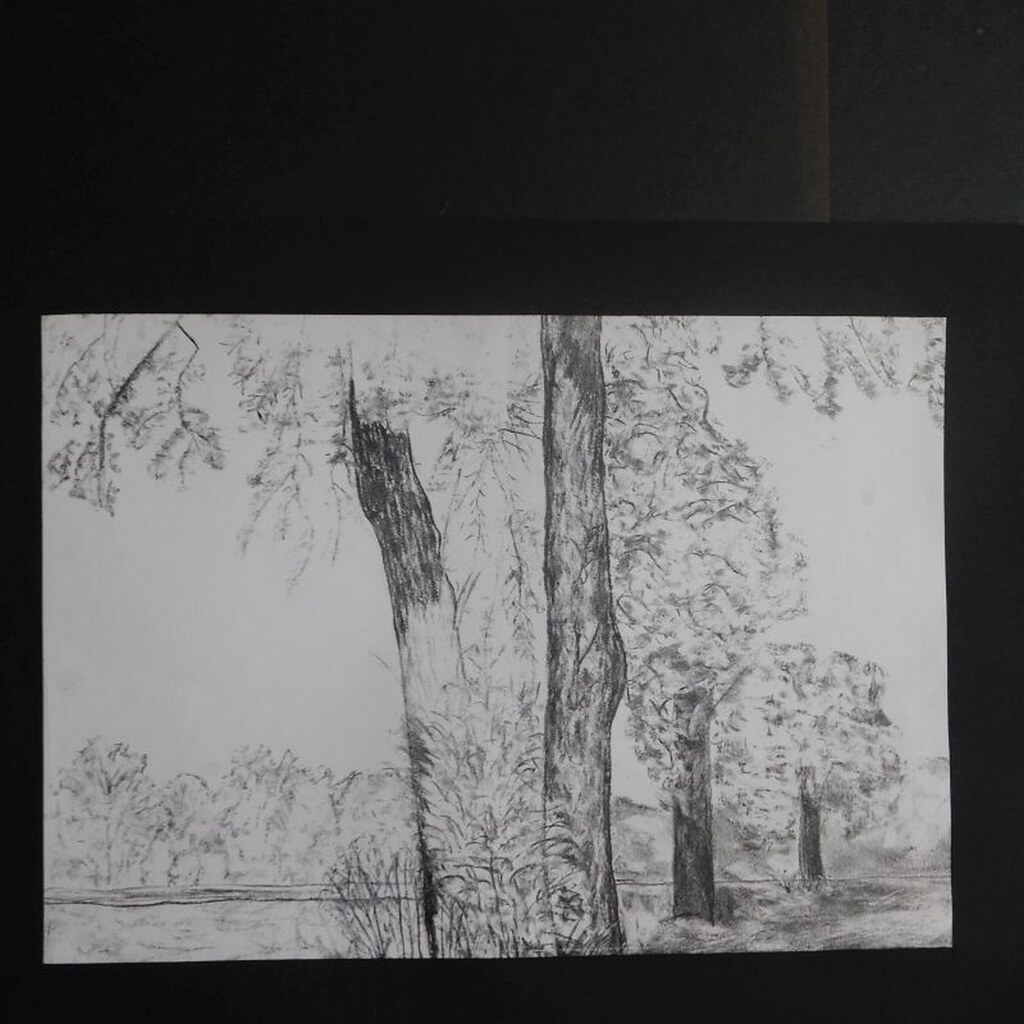This black and white photograph captures a detailed charcoal drawing of a landscape scene on white paper, likely from a sketchbook or printer paper. The drawing includes a variety of trees prominently featured in the foreground, showcasing tall trunks with most of their foliage high up, leaving sparse greenery at lower levels. Among these, two large trees stand out, accompanied by fluffy shrubs and smaller grasses at their bases. The scene extends into a background where a mix of other trees, including some coniferous trees and possibly a mix of hogweed and shrubs, contribute to the depth of the drawing. Some branches hang down, adding texture to the upper part of the foreground. The horizon line is defined by another row of trees with fuller foliage lower on their trunks. Notable are the smudges and fingerprints visible on the paper, hinting at the artist’s hands-on techniques. The drawing, rich with shading and varying textures, gives an impression of either a lake with waves or a field with blades of grass or wheat. The detailed depiction resides on what appears to be a black desk, enhancing its grayscale tones.